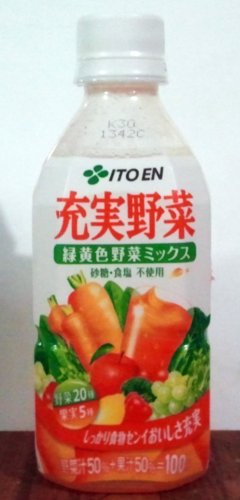The image depicts a contemporary photograph oriented in portrait mode, emphasizing its vertical alignment. The subject of the image is a bottle of juice, with a prominent white label that features splashes of green and red. The product appears to be of Chinese origin, as indicated by the Chinese characters displayed in red near the top of the label. Above these characters, the brand name "Ito En" is elegantly written in black manuscript letters, accompanied by a small green flower symbol. 

Below the red characters, there is an additional row of green and white characters. Centered on the label is an illustrative depiction of various fruits and vegetables, including carrots, spinach, tomatoes, and grapes, suggesting that the juice is a blend of both fruits and vegetables, similar to a V8 beverage. The lower portion of the label details the product's weight. The bottle itself is sealed with a white cap, adding to the clean and fresh presentation of the juice.